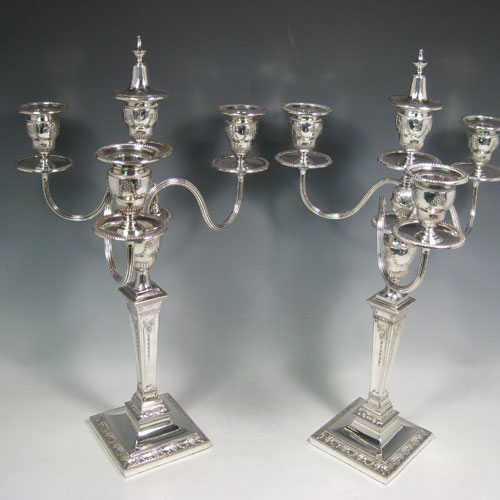This color photograph features two intricately designed silver candelabras, set against a light gray background that darkens towards the top, giving it a subtle gradient effect. Each candelabra showcases a wide, square base which transitions smoothly into a smaller pedestal. From this base, a tapered stem rises elegantly to support the main structure. The design includes four ornate, wavy arms that extend outwards, each ending in a circular candle holder shaped like a cup. Positioned behind these arms is a trio of additional candle holders, one situated at each end and one in the center, creating a distinctive row behind the front holders. Topping off the candelabras, at their very center, is a pointed silver tower that adds a sophisticated touch. The silver of the candelabras subtly reflects the light, adding dimension and a mirror effect to the image.